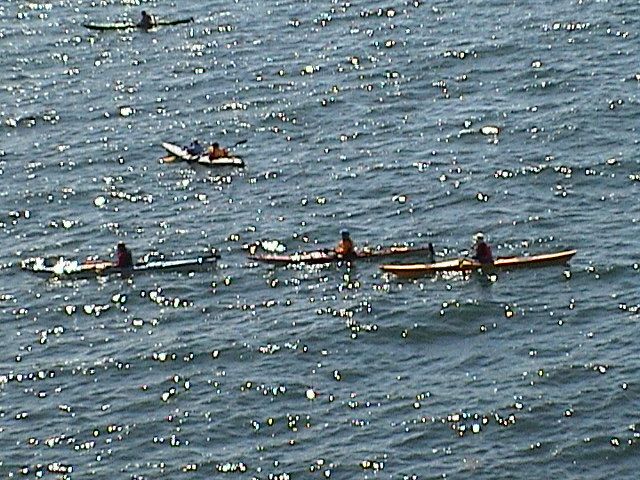This photograph, taken from a distance and looking down, captures a group of people canoeing on a bluish body of water. The image is somewhat blurry, which makes it difficult to distinguish the details of the people or what they are wearing. There are five sleek, elongated canoes scattered across the water. In the foreground, slightly below the center of the image, three canoes are closely grouped together. Above them, towards the left of center, a fourth canoe is approaching, containing two people. In the upper right corner, a fifth canoe with one person is visible. The surface of the water appears slightly rough, with ripples and white foam dotting the scene, adding texture to the blue expanse. Overall, the image captures the dynamic nature of the canoeists as they row with long paddles, emphasizing the activity and the natural setting.